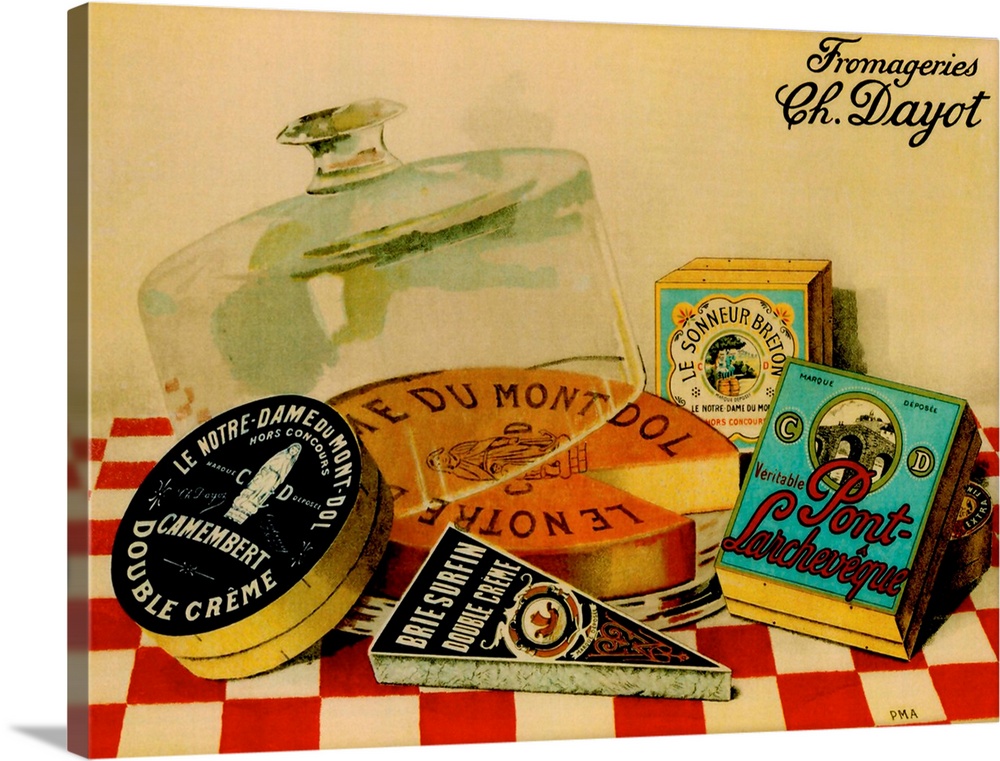The image depicts a detailed drawing reminiscent of an advertisement or a billboard, set against a tan background transitioning to a red and white checkered floor towards the bottom. Centrally, there is a selection of French cheeses. A large, round cheese occupies the middle with a slice missing and labeled "Dew Mont D'ol" in French script, partially covered by a tilted glass dome typically used for cakes. To the left, there's a triangular double cream cheese, probably brie, and next to it, what appears to be a Camembert cheese, also double cream. On the right, a cheese with a blue cover is present, while in the background, another item with a yellow cover can be seen. The top right corner of the image features the text "Fromageries Ch. Dayot" in elegant black script. Additional elements in the scene include a small tin with a black-and-white lid on the left and two boxes along with a spool of thread on the right, all resting on the checkered tablecloth.